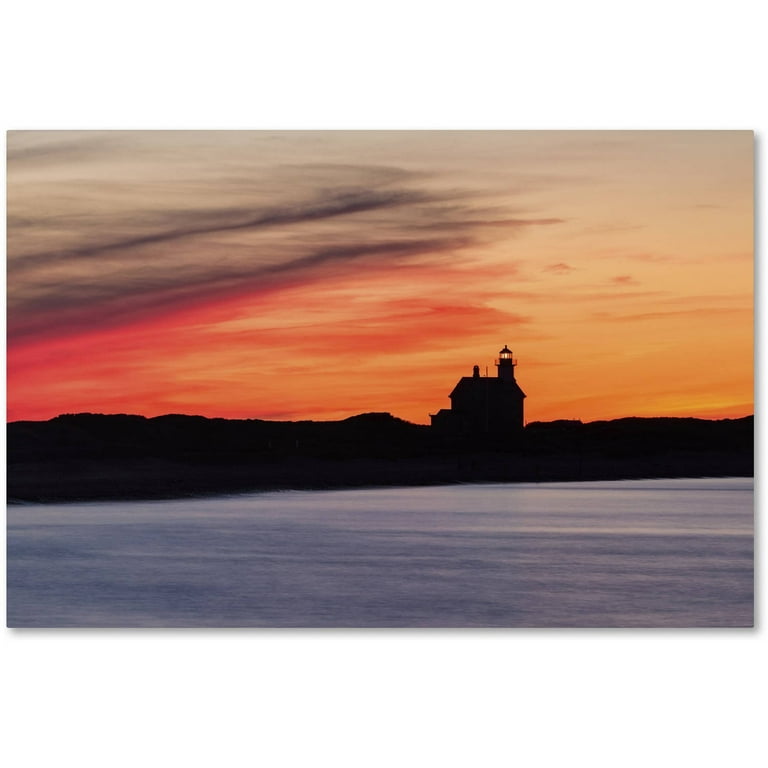A visually stunning image captures a picturesque lighthouse at sunset, though it's hard to discern if it's a photograph or a painting. Dominating the lower third of the composition, the steel-blue and flint-colored sea stretches calmly, save for a few delicate white lines mimicking gentle waves. Silhouetted land cuts across just above the water, with the lighthouse standing prominently in the right third of the frame. The sky above is a tapestry of colors, transitioning from a pale grayish-yellow at the very top to deep, fiery oranges and reds closer to the horizon, tinted with dark gray clouds. Golden and yellow streaks from the last rays of the sun shoot off to the right, completing this captivating sunset scene over the serene waters.